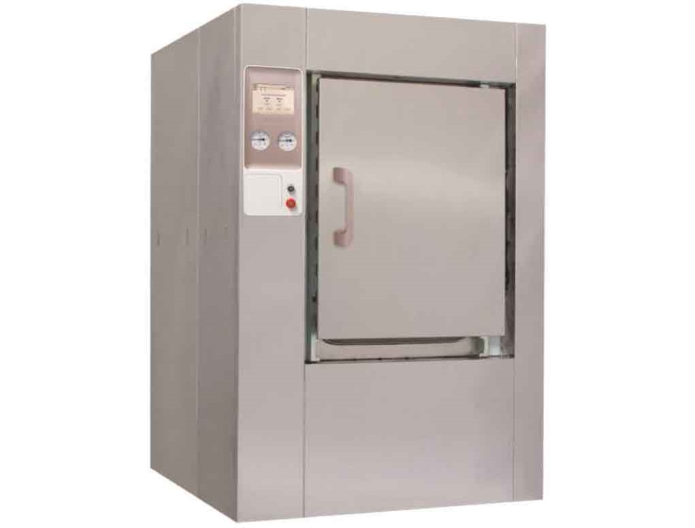This image features a steel rectangular box with a dull gray color and prominent angular edges. The box has a vertically oriented door on the front, which is equipped with a long handle protruding outward in a backward C shape. On the upper left side of the box, there are two dial indicators with needle hands, presumably to measure internal conditions such as temperature or pressure. Directly below these dials is a small panel, which appears to house two buttons—one black and one red, the red being larger. Above the dials and panel, there's a white label with black text, though its content is unreadable. The box is likely some kind of pressurized or temperature-controlled cabinet, possibly a cooler, as suggested by the presence of a black seal designed to maintain the internal environment. The background of the image is entirely white, giving no additional context. The entire assembly is estimated to be approximately three feet tall.